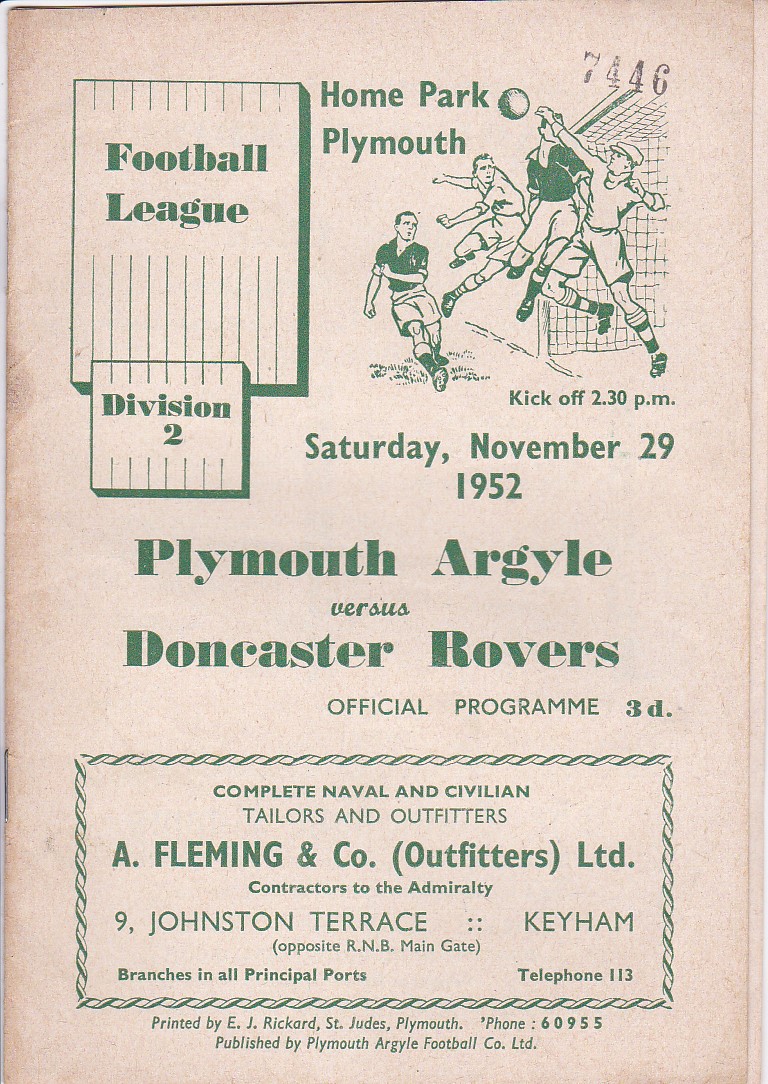The image is an old advertisement, possibly for a football game, appearing on what looks like an aged paper. The prominent text on the page reads "Home Park Plymouth Football League, Division II," with details of a match scheduled for "Saturday, November 29, 1952" and a kickoff time of "2:30 p.m." The main event features "Plymouth Argyle versus Doncaster Rovers," described as the "official program." 

In the top right corner, there's a small image showing two teams in action, with one team in dark jerseys and the other in white. Below the event information, additional content highlights "A Fleming and Co. Outfitters Limited," noted as contractors to the Admiralty, located at "9 Johnson Terrace," and possibly in "Keyham," with branches in all principal ports and a phone number "113." Further down, it says "Printed by EJ Rickard, St. Jude's, Plymouth," providing another contact number, and states that the publication is "Published by Plymouth Argyle Football Co. Limited."